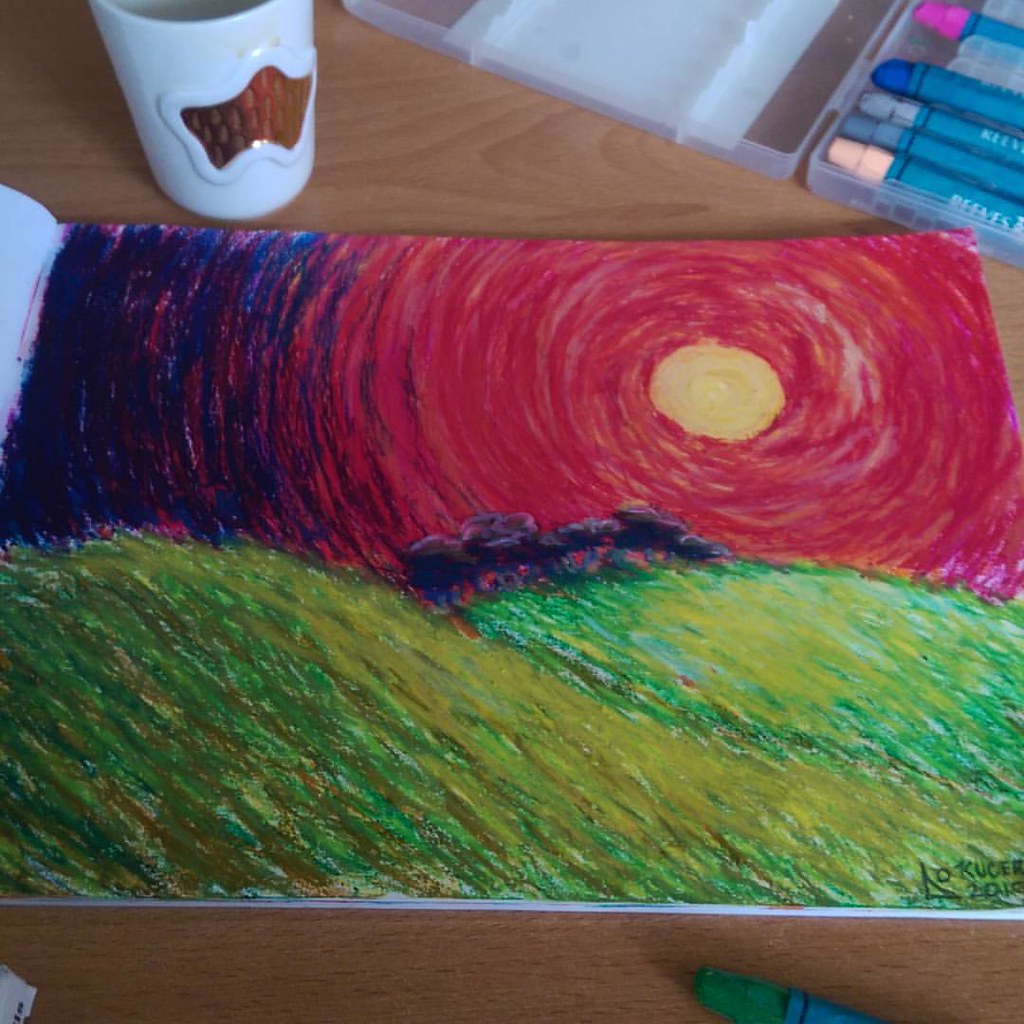On a sturdy brown wooden desk sits a meticulously painted reproduction of Vincent van Gogh's "Starry Night." At the top of the desk, a single green wax crayon lies casually, hinting at recent artistic endeavors. In the foreground, an open pack of wax crayons reveals a few missing colors, suggesting they have been used. Adjacent to the crayons, a white mug adorned with a golden star stands empty, its previous contents likely consumed. The painting on the desk is signed at the bottom with the name "Kucer" and a partially visible date that appears to be either 2019 or 2010, though the full year is obscured.